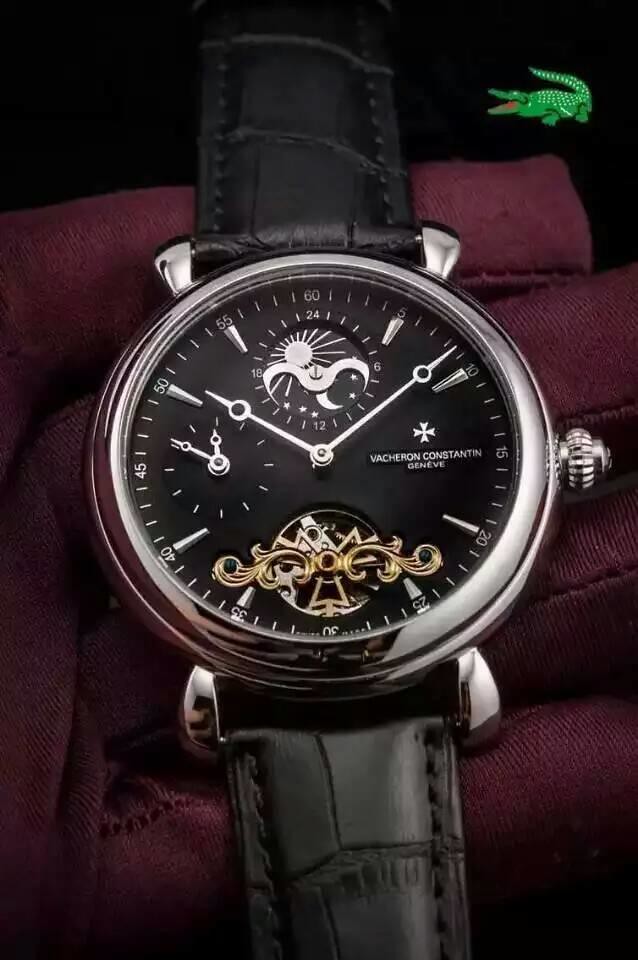The close-up color photograph showcases a luxurious wristwatch with a polished silver edge and intricate details. The watch features a black face adorned with two secondary dials at the top and bottom, and an additional small sub-dial to the left. Numerous pointed markers replace traditional numerals around the watch face. The watch hands and a circular motif, resembling a mountain and sun at the top of the dial, are both silver. At the bottom of the watch face, there's a gold swirling design within a circle. A silver logo on the right side reads "Vacheron Constantin Geneve." The black leather strap with detailed stitching gracefully attaches to the watch, and on the side, a knob with indented grips adds functionality.

The timepiece is artistically placed on a rich, burgundy velvet or satin cushion that is crumpled, adding to the sophisticated presentation. The background remains a stark black, allowing the watch and its cushion to stand out prominently. In the upper right corner of the image, a bright green Lacoste alligator logo overlays the scene. The alligator, with its mouth open, displaying a vivid red interior, appears almost like a watermark, possibly suggesting a professional touch or branding. Additionally, a maroon-gloved hand with thick stitching grips the watch, adding a touch of elegance to the overall composition.